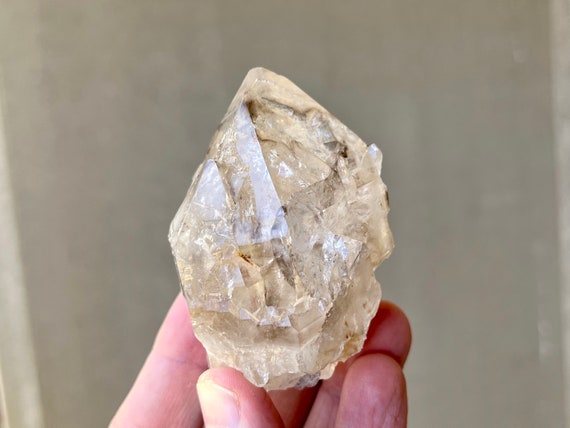The close-up image features the tips of someone's fingers holding a large, jagged crystal that appears almost translucent with some gray and black streaks and specks of beige towards the bottom. The crystal, which may be quartz, shows complex details including rough and smooth areas. The smoother, pointy tip of the crystal glistens under a light, creating a white sheen and faint reflections that add depth to its silvery-white and clear appearance. The person, likely described as a white male based on their skin tone and nail appearance, holds the crystal with both hands, thumb touching the lower left corner, and other fingers – notably the thumb, pinky, and ring finger – visibly positioned to support the crystal from its sides. The background is blurred and indistinct, resembling a light gray wall, ensuring that the focus remains on the intricately detailed crystal and the careful grip of the holder's fingers.